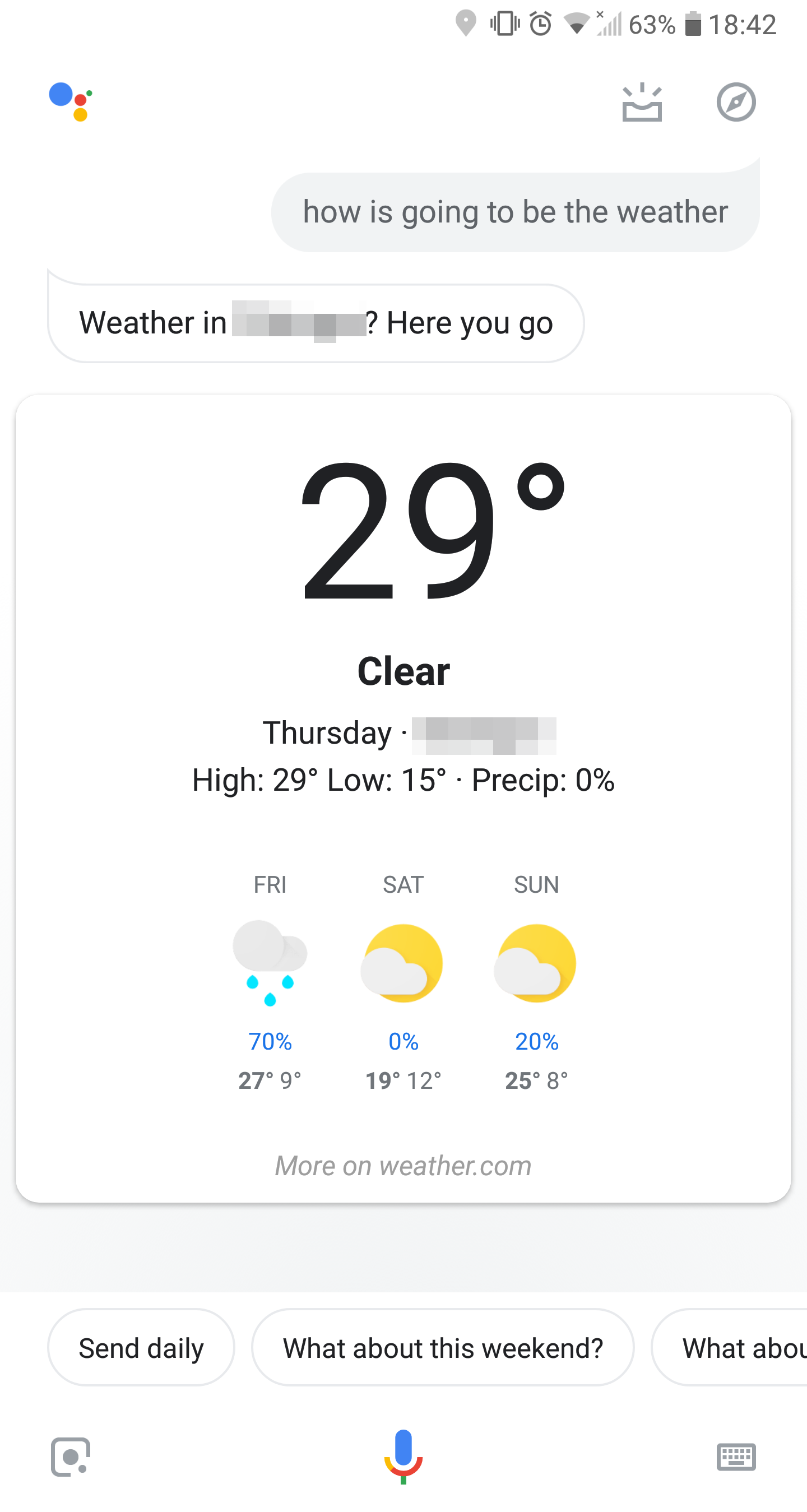The image showcases a mobile app developed by Google, presenting the current weather conditions. The screen is filled with various indicators and icons. In the upper left corner, a multi-colored arrangement of blue, red, orange, and green circles is displayed. On the upper right, standard mobile icons indicate the device’s status: location services, vibration, alarm set, Wi-Fi connection, and cellular signal strength. The battery is at 63%, with a time display showing 18:42 (6:42 PM). Directly below these icons, the user’s inbox and a navigational compass star are visible.

Following this, there is a somewhat awkwardly phrased text: "How is going to be the weather." This is succeeded by an inquiry and response: "Weather in [blurred location]? Here you go, 29 degrees, clear, Thursday."

In the center section, a detailed forecast is provided, specifying a high of 29 degrees and a low of 15 degrees, with 0% precipitation for the day. Further down, the forecast extends to the coming days:

- **Friday:** 70% chance of snow, indicated by a grey cloud and blue rain dots icon. The temperature high is 27 degrees, with a low of 9 degrees.
- **Saturday:** Displays a slightly cloudy yet sunny icon, with no precipitation expected. The high will be 19 degrees, and the low 12 degrees.
- **Sunday:** Shows a sun with partial cloud cover icon, a 20% chance of precipitation. The high is expected to be 25 degrees, and the low 8 degrees.